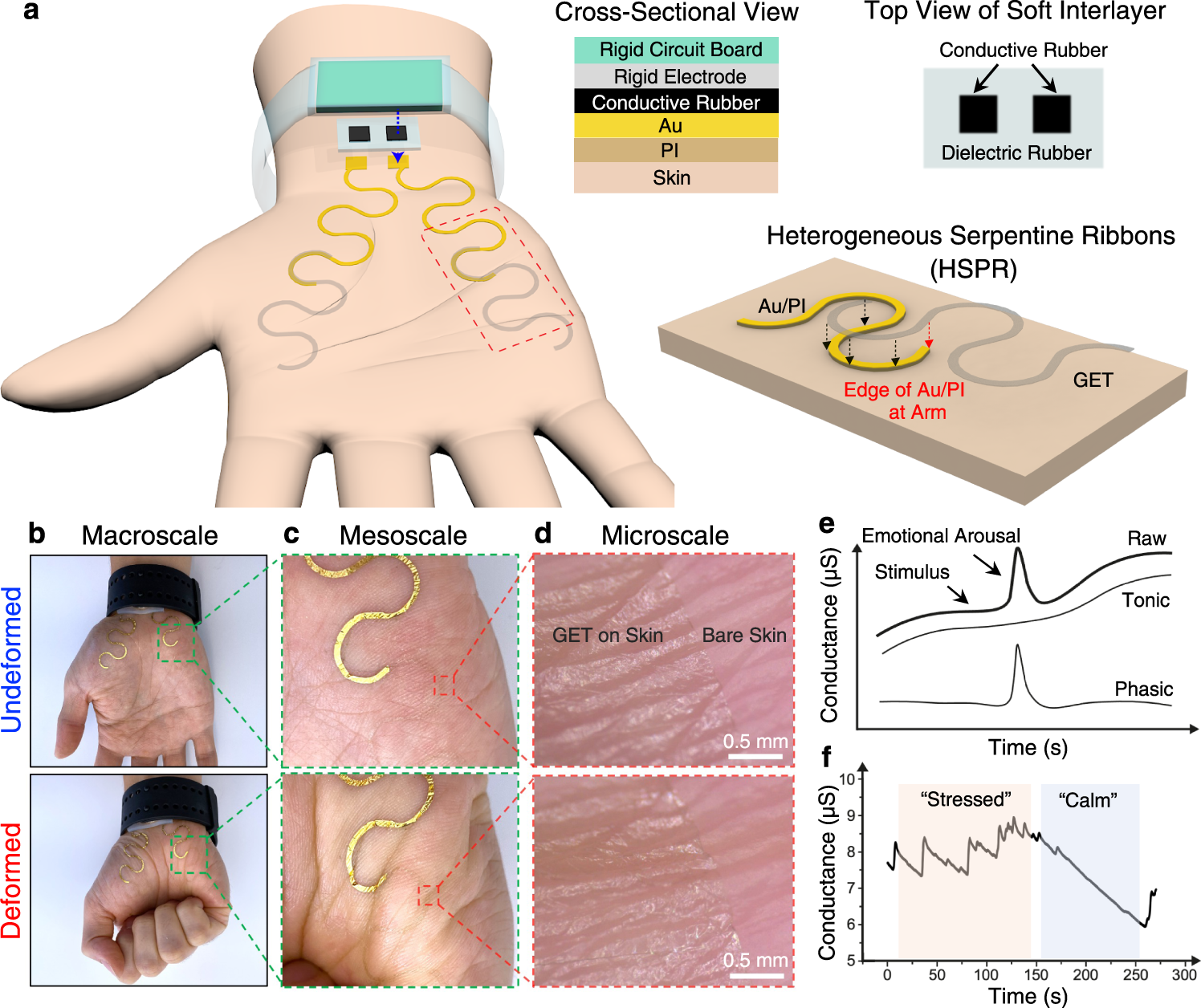This textbook page presents a detailed diagram and analysis of a sensor-equipped hand, illustrating various scales and emotional arousal metrics. At the top left (labeled A), an artificial rendering of an outstretched hand wearing a Fitbit-like bracelet displays squiggly yellow and gray lines emanating from a rectangular device on the wrist, indicating the heterogeneous serpentine ribbons (HSPR) beneath the skin. A key beside the hand delineates components such as the rigid circuit board, rigid electrode, conductive rubber, AU, PI, and skin.

Beneath this, categorized under B, six sequential photographs illustrate the hand from a macro to a microscale view. The initially undeformed hand transitions to a deformed hand in a fist, each stage meticulously detailing the skin texture.

Adjacent to these images are explanations and top views of soft interlayers, providing insights into the internal workings of the sensor. Sections labeled C and D elaborate on the HSPR, detailing intersections and material compositions.

The lower right section (labeled E and F) features graphs plotting conductance over time, correlated with emotional arousal states—stressed and calm—and unspecified stimuli. These graphs provide a quantitative analysis of the sensor’s measurements, linking physical hand movements to emotional states. The photograph and diagram collectively offer a comprehensive study of the sensor's capabilities and its applications in monitoring physiological and emotional changes.